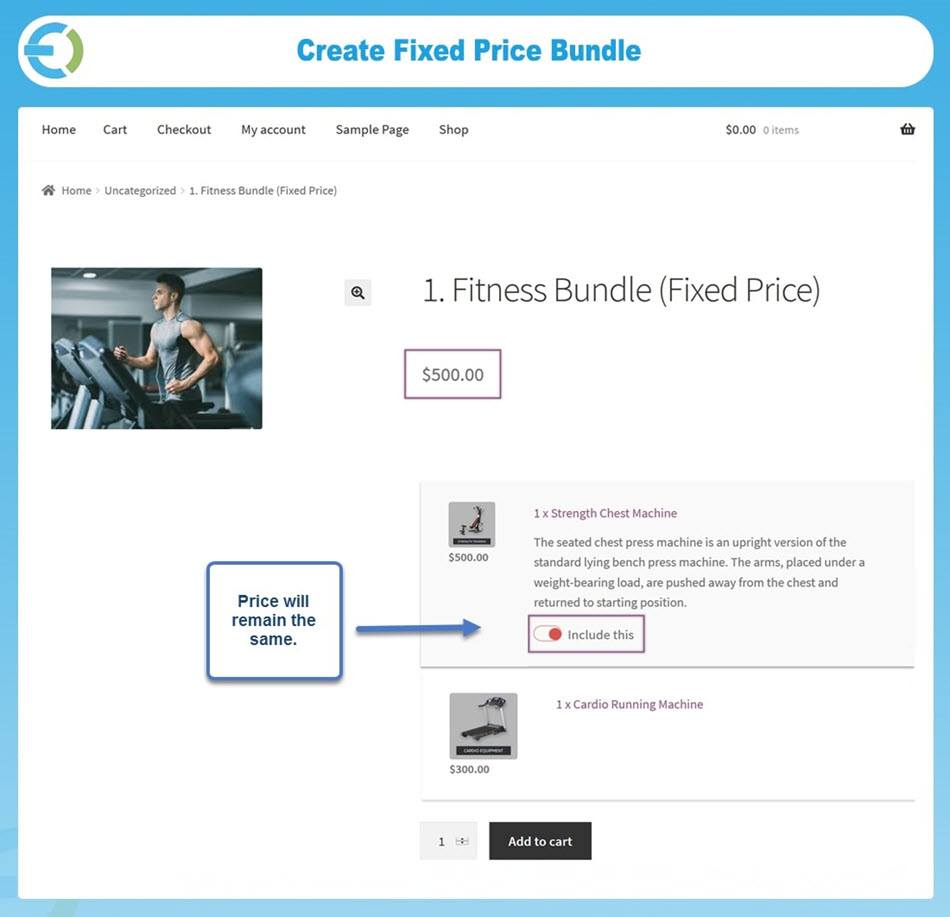In the image, the header prominently displays the text "Create Fixed Price Bundle" in blue, positioned at the center top. On the top left corner, there's a circular logo divided into blue on the left and green on the right. Below the header, there is a horizontal menu bar listing several categories: Home, Carts, Checkout, My Account, Sample Page, and Shop. Toward the right of the menu bar is a blank space, followed by the text "$0.00, zero items," and an adjacent shopping cart icon.

Dominating the center of the image is the text "1 Fitness Bundle" followed by "Fixed Price." Directly beneath, a purple, squared box highlights the price "$500." To the left of this price box, there is an image in another squared box depicting a person running on a treadmill. This individual has a light skin tone, short black hair, and is wearing a gray athletic shirt.

In the lower right section of the image are two smaller boxed sections. The top box, outlined in purple, reads "1x Strength Chest Machine" and contains a small image of the chest machine. Below it, the bottom box states "Cardio Running Machine" and also includes a small image of the running machine on the left.